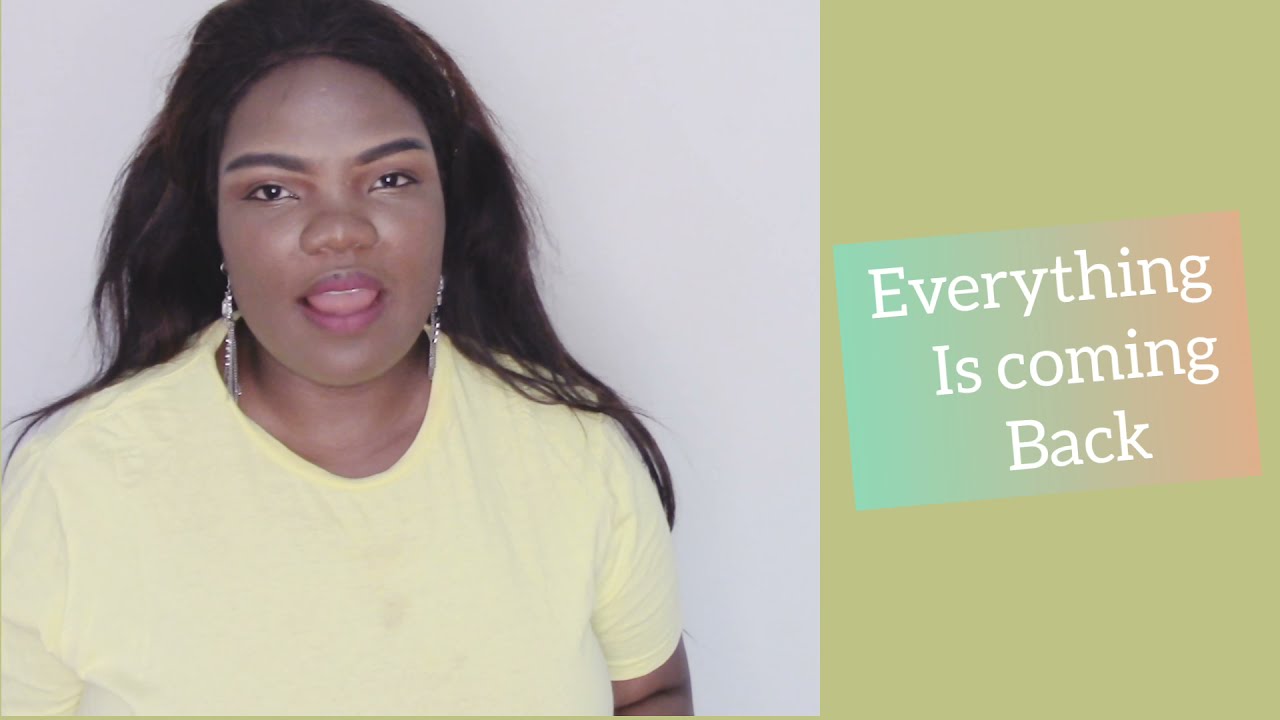The image is a rectangular composition split into two distinct sections. On the left side, occupying approximately two-thirds to three-quarters of the space, there is a young African-American woman. She stands against a light gray or whitish background, facing forward with her mouth slightly open as if she's speaking. She has long, straight dark hair that drapes over her shoulders, pulled back from her forehead with a headband or similar accessory. Her attire includes a short-sleeved yellow t-shirt, and she sports long, dangly earrings that sparkle. Her arms appear to be folded up, contributing to the sense that she is addressing someone.

On the right side, the remaining one-third of the image features a solid light sage green or olive green background. Within this green section is a smaller, inner rectangle with a gradient fill transitioning from teal on the left to light pink on the right. This rectangle contains white text that reads, "Everything is coming back," suggesting a possible promotional message or theme. The overall layout and design imply that this could be an advertisement or a slide from a presentation or video, with the woman prominently positioned to draw viewer attention while the text on the right conveys the core message.